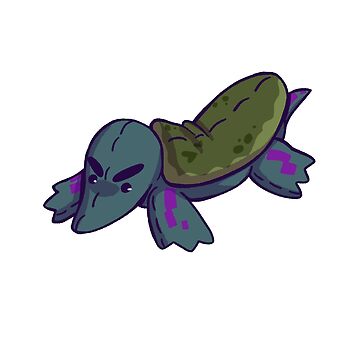This detailed cartoon image features a grumpy, stuffed platypus-like creature with a blend of characteristics that suggest it might also be a turtle or a dinosaur. The figure stands against a completely white background, emphasizing its features. It has a single stitched seam running from the top of its nose down its back, reinforcing the stuffed toy appearance. The body is dark green, complemented by a soft, oval-shaped pad on its back with black lines running through the middle, resembling a shell or a leaf.

The creature's head, adorned with thick black eyebrows and small beady eyes with tiny white pupils, faces the lower left corner of the image. Its expression is one of visible discontent. A small shadow on top of its nose gives the impression it's slightly bent upwards. It has four paddle-like legs with purple spots on each, and a short pointed tail with a hint of purple too. The detailed though simple art style, combined with whimsical color choices like the olive green pad on its back, gives the overall impression of a well-loved, sewn toy.